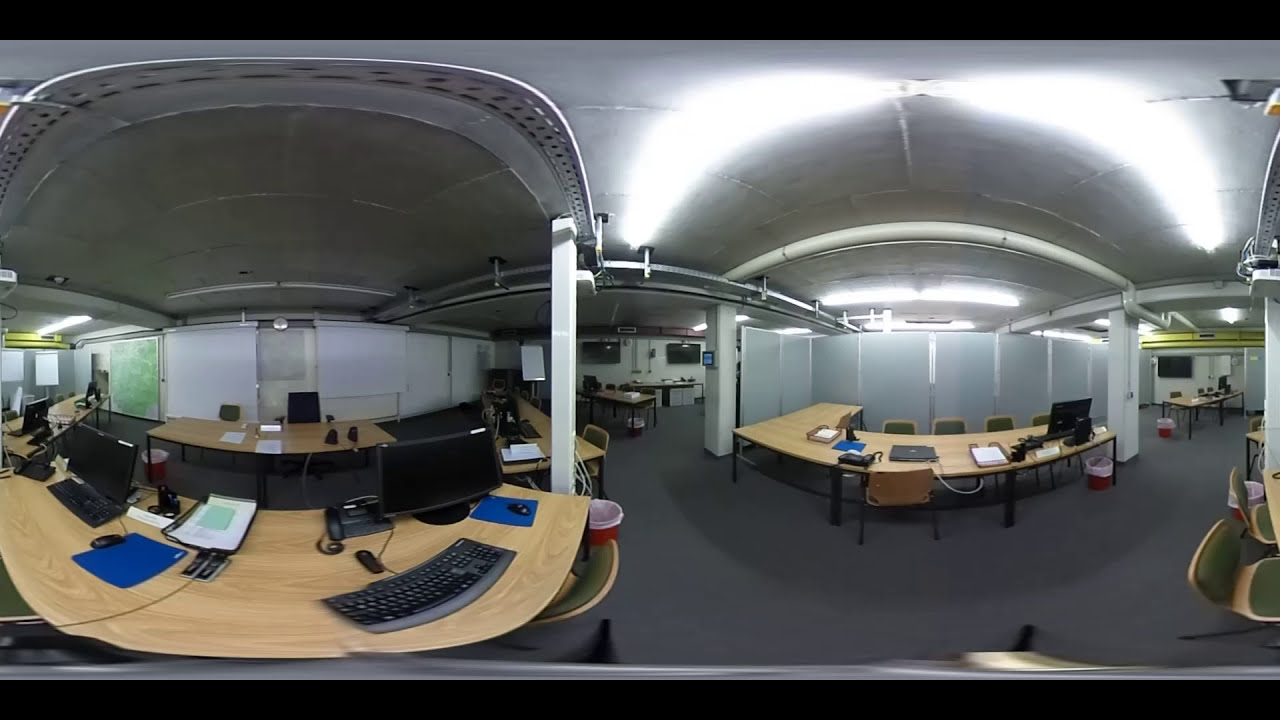The image depicts a well-lit, spacious office area characterized by an array of light brown, sandy-colored desks with various configurations, including several L-shaped and rectangular tables. Each desk is equipped with computer screens, keyboards, and chairs. On the left side, there is an L-shaped desk featuring four computer monitors, with additional tables behind it. The right side showcases another L-shaped desk with a laptop and a black computer monitor, along with numerous chairs aligned along its length. The office is lined with white walls, dotted with white pillars, and has a darker gray ceiling with long rectangular lights. TV monitors are mounted on the walls throughout the space, enhancing the modern ambiance. The floor is gray, complementing the overall neutral color scheme of the office.